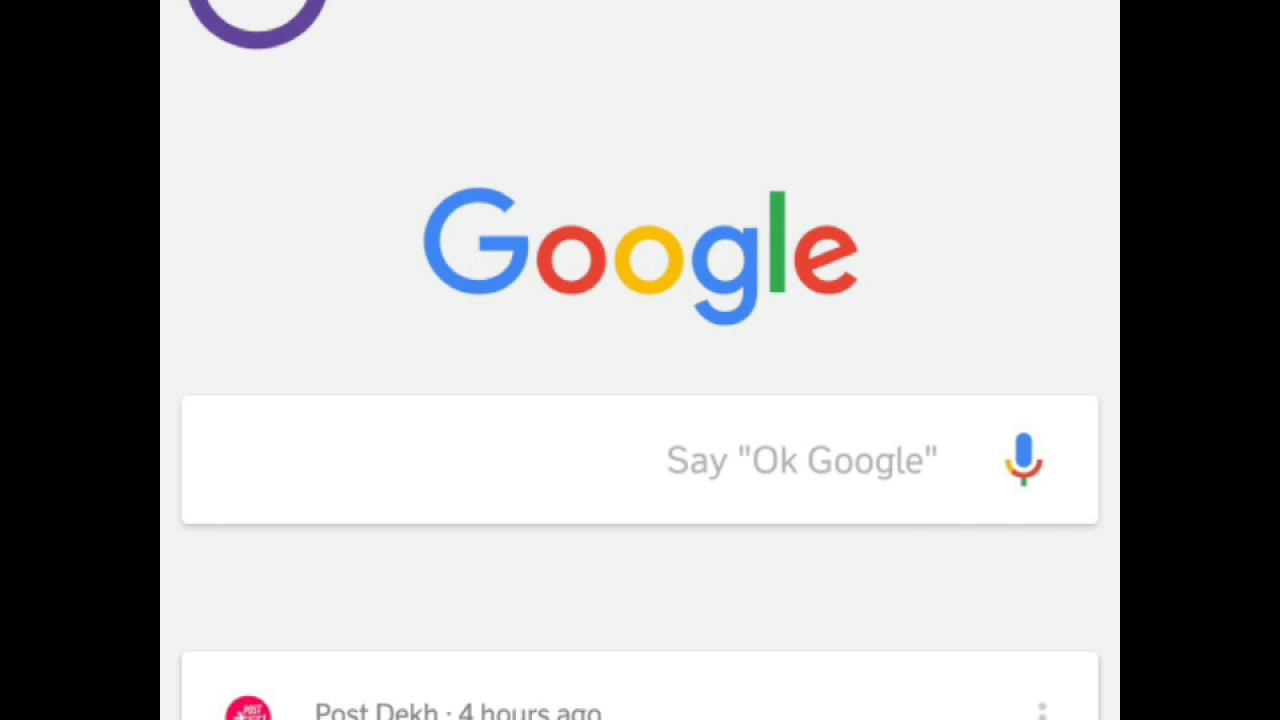A detailed screenshot of a Google search page, captured most likely from a cell phone due to its portrait orientation and similar dimensions. The landscape-shaped photo overall is much wider than it is tall, bordered by thin vertical black rectangles on the right and left, each accounting for roughly 15% of the screen width.

At the center of the image, a square-shaped gray background dominates. At the top left, a purple semicircle intrudes slightly. Centrally positioned, the iconic Google logo stands out, with "Google" spelled in a distinctive sequence: a capital 'G' in blue, an 'o' in red, another 'o' in yellow, a 'g' in blue, an 'l' in green, and a sideways 'e' in red.

Below the logo, a white search box invites interaction. Inside the box is a prompt in gray font reading, "Say 'OK Google,'" accompanied by a multicolored microphone icon comprising blue, yellow, red, and green hues. Below this search box, the gray background resumes, ending with a text bubble that appears to be in a foreign language.

Further down, a pink circular icon features a recent interaction, stating, "Post your DEKH four hours ago."